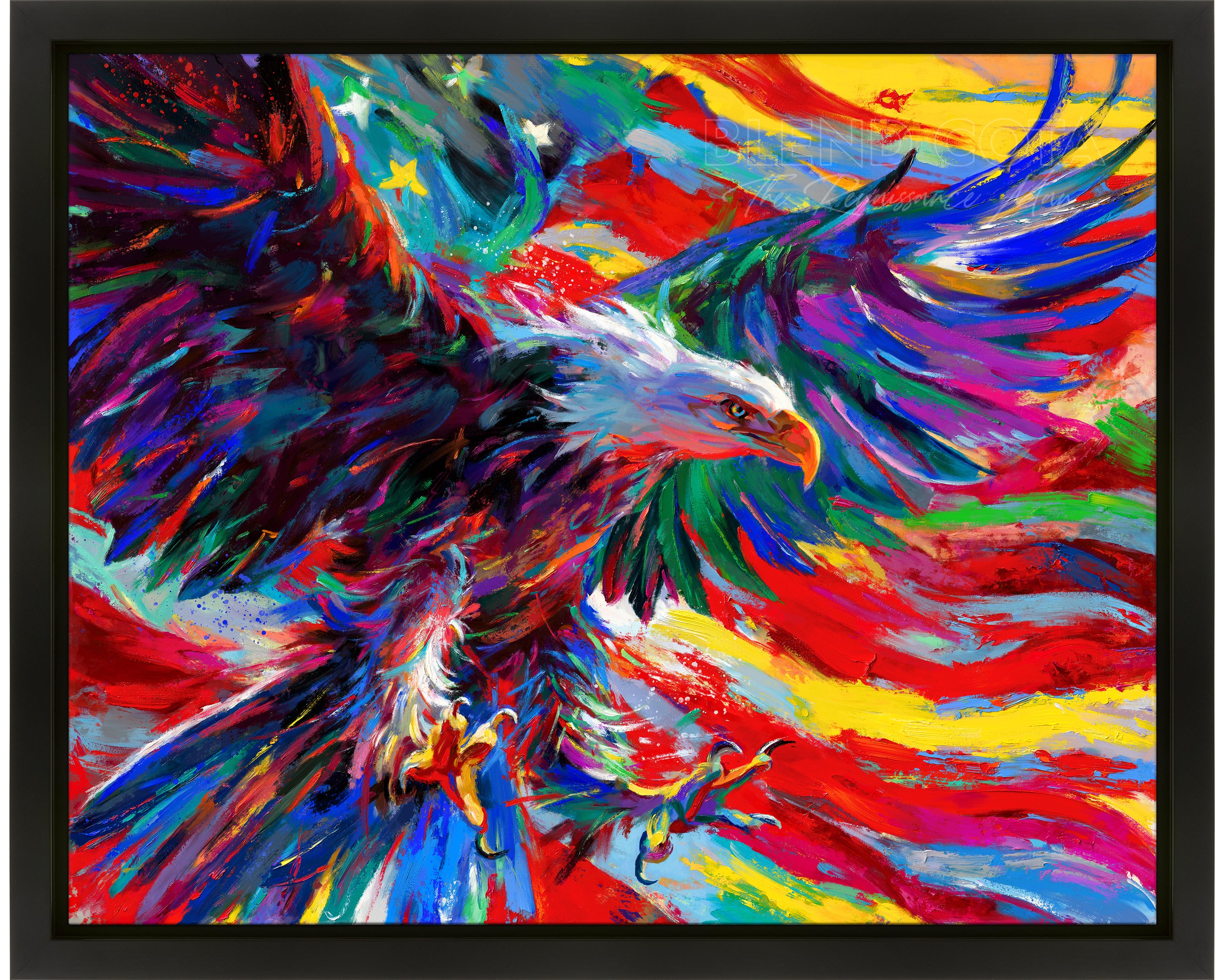This image showcases a square, psychedelic-style painting of a bald eagle in flight, framed by a black border. The eagle's wings are outspread, and its talons are extended as if hunting. The head of the eagle, predominantly white, faces to the right. The body and wings are adorned with an array of colors, including black, green, blue, pink, and shades of purple, blue, and green. The wings and tail feature intricate blends of these colors, giving the painting a fluid, almost surreal appearance.

In the background, there is an abstract, stylized rendition of the American flag. The top center shows a blue and green field with four white and yellow stars, while the wavy stripes are rendered in an unconventional palette of red, yellow, blue, teal, and green. These stripes flow dynamically across the image, enhancing the sense of motion and blending seamlessly with the red marks and strokes of yellow and blue on the bottom right. The overall effect is one of vibrant, harmonious chaos, capturing both the majesty of the eagle and the spirit of the American flag in a unique and visually striking manner.